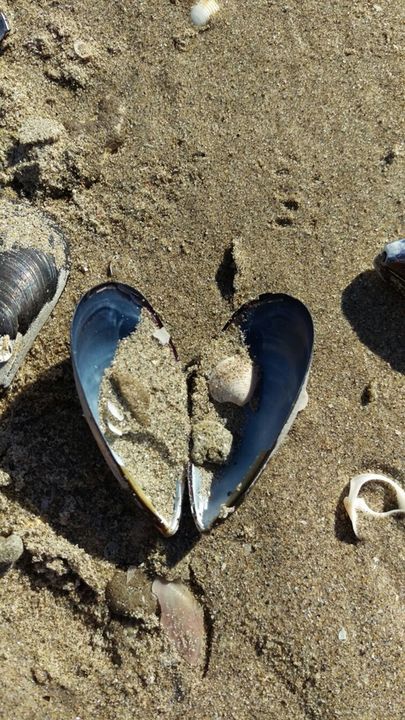This is a color photograph in portrait orientation, depicting a detailed scene of wet, light beige sand at the beach, likely near the water. At the center of the image lies an opened mollusk shell, beautifully showcasing a heart shape with its two halves. The inner part of the shell is a striking blue, bordered by black edges, and it contains a smaller shell inside, along with some sand. Surrounding this central shell is an array of other shells and fragments: a black shell on the left, a partly buried shell tip on the right, a broken white shell below, and various other smaller shells scattered throughout. The sand is interspersed with very small, light brown stones, and tiny air bubbles emerge from its surface. The scene is bathed in sunlight, casting subtle shadows and adding depth to the natural composition.